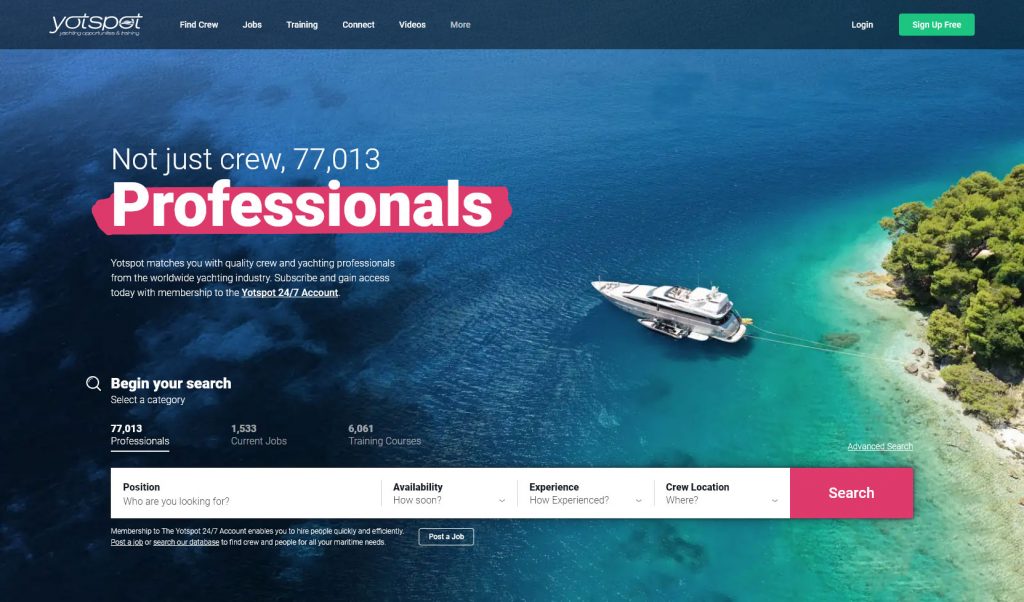The image depicts the homepage of the Yotspot website, spelled Y-O-T-S-P-O-T. In the top left corner, situated on a blue panel that stretches across the screen, the Yotspot name and logo are prominently displayed. Various headings are visible on this blue panel, including "Find Crew," "Jobs," "Streaming," "Connect," and "Videos." On the far right side, there are links for "Login" and signing up "For Free," the latter accompanied by a clickable green button.

Beneath the blue panel, a large, striking image of a yacht moored on what appears to be an island or beach, surrounded by the sea, captures the viewer's attention. To the left of this image, the site highlights its extensive network with the phrase "Not Just Crew – 77,013 Professionals" written in bold white font and underlined with a pink marker, drawing immediate focus.

Further down, the site elaborates on its core function, stating that Yotspot connects users with quality crew and yachting professionals from the global yachting industry. Below this information, there is a search dialogue box where users can input criteria such as position, availability, experience, and crew. To initiate the search, users can click on a prominently placed pink search button.